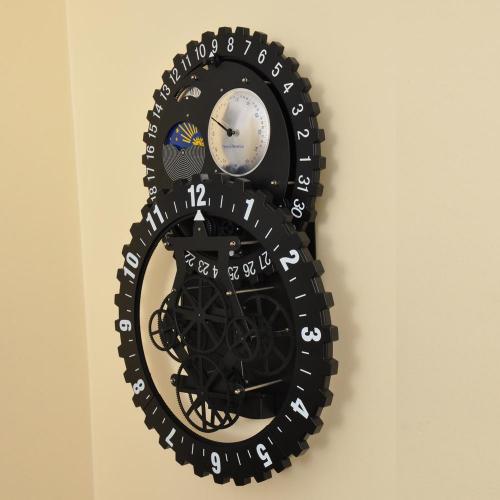This photograph captures a highly intricate clock mounted at the corner where two beige walls converge. The clock features a uniquely mechanical design, with an upper circular component displaying the numbers 1 through 12, akin to a standard clock face. This circle appears to float above a larger, lower circle, which showcases numbers ranging from 1 to 31, possibly indicating days of the month. Various dials and smaller wheels are integrated into the structure, adding complexity to its appearance. A European Union flag is also depicted within the composition, enhancing its distinctive aesthetic. The clock is partially open, revealing a fascinating array of gears and mechanisms, offering a rare glimpse into its inner workings. This split-open design adds to the allure of the piece, blending functionality with a display of intricate craftsmanship.